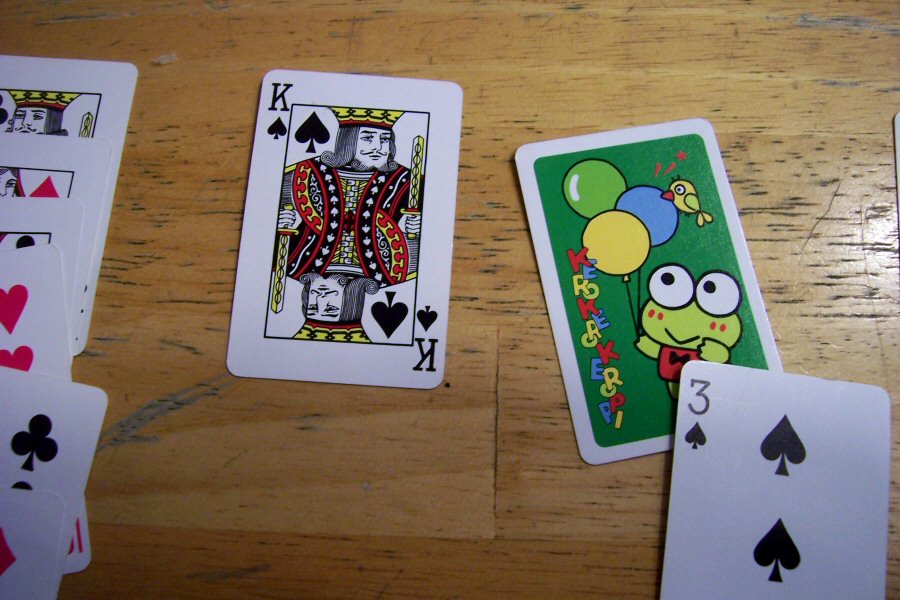A well-worn pine tabletop, with its grain and scratches telling tales of years of use, serves as the setting for a spread of playing cards. The surface, though uneven and imperfect, exudes character. In the foreground, the King of Spades sits solemnly, separate from the rest. Beside it, a smaller, unique card features a whimsical frog cartoon. The cheerful amphibian, set against a vibrant green background, grips three colorful balloons—two shades of green and one blue. Encircling the frog, the text "k-k-k-k-k-k-k-k-k-k-k-k-k-k-k-k-k-k" humorously mimics the creature's repetitive croak, adding a playful touch to the scene. The card's distinct size and unconventional design contrast with the standard deck, hinting at its special, possibly sentimental, significance.